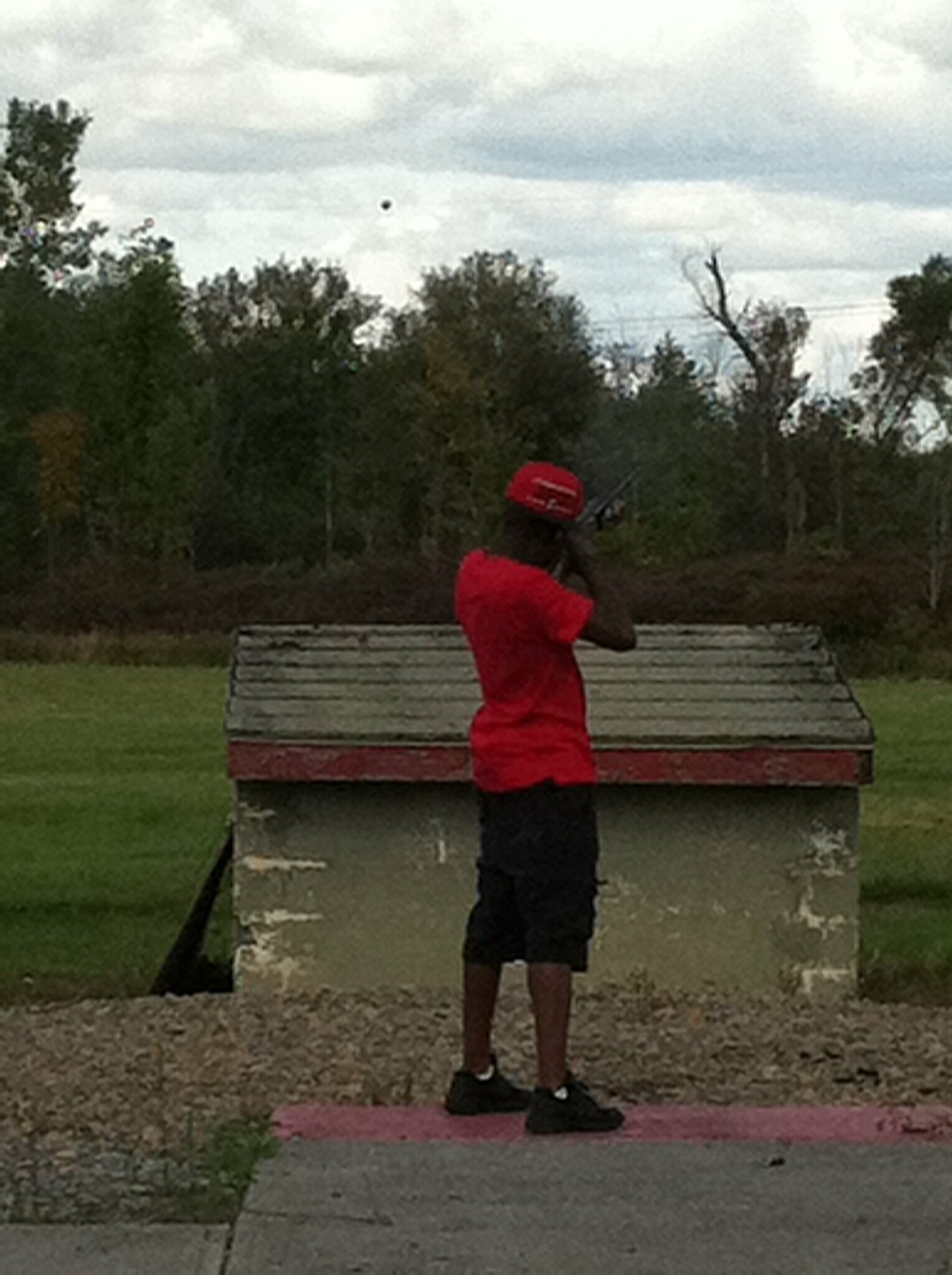A photo captures a dark-skinned male standing on a concrete pad amid an outdoor setting. The man, dressed in a red short-sleeved t-shirt, black knee-length shorts, and dark running shoes, also wears a red roundish cap. He is holding a rifle, which is pointed away from the viewer, aiming towards an area with trees in the distance, potentially indicating he is about to shoot at something. Positioned ahead of him on lower ground is a concrete shed with a dark grey shingled roof. The roof's edge aligns with his shoulder height, and the shed is surrounded by wood chips, gravel, and grass, with a wider field bordered by numerous trees extending in the background. The sky overhead appears to be cloudy.